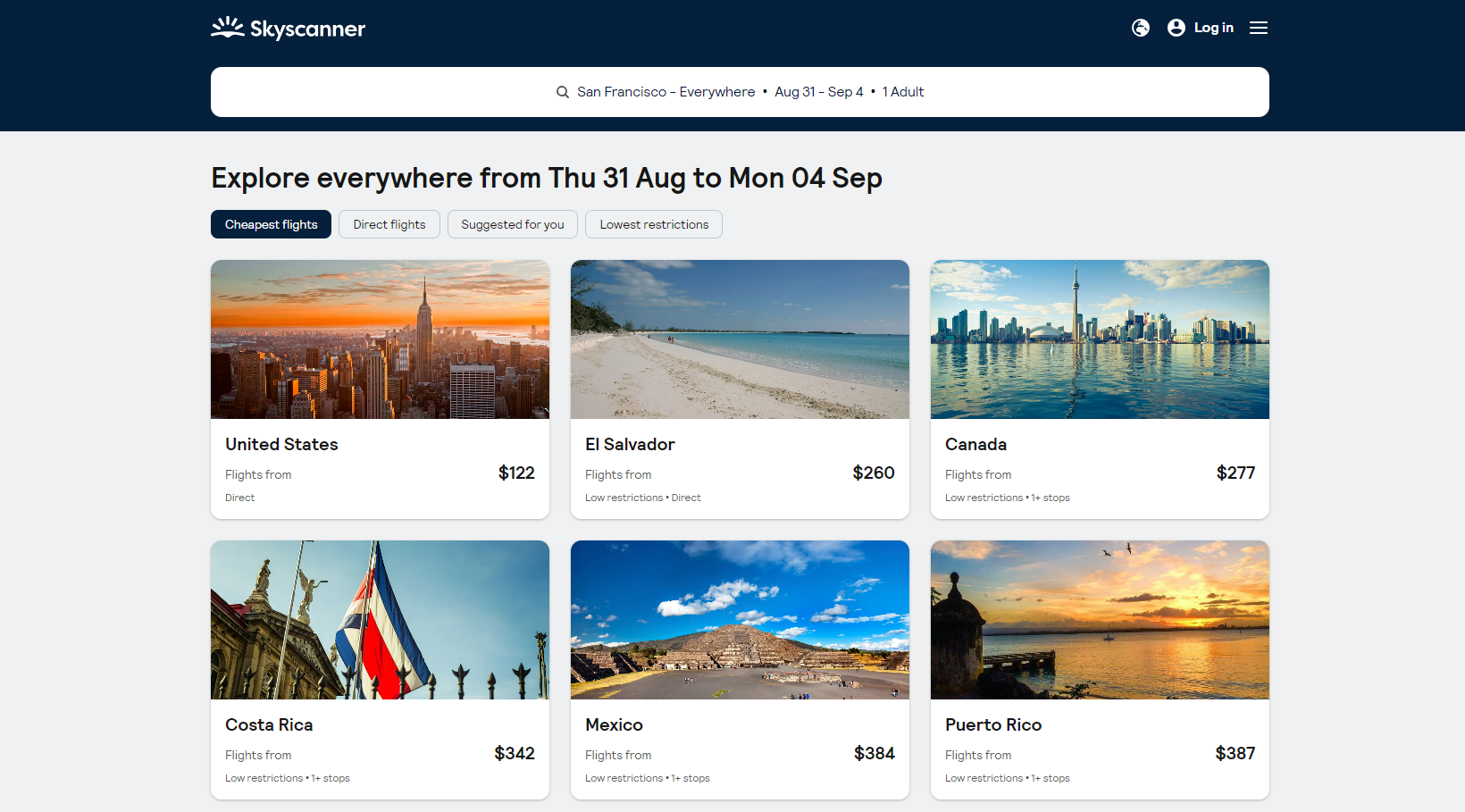This image is a cropped screenshot of the Skyscanner website. The header, which is dark blue, prominently features the Skyscanner logo on the top left. Beneath the header runs an extensive search bar with the input text stating "San Francisco, everywhere, October 31st to September 4th, one adult." The body of the website below the header has a gray background. At the top left of this section, the text reads "Explore everywhere from Thursday 31st August to Monday 4th September."

Below this introductory text, there are two rows of flight deal thumbnails. The first row displays three destinations:
1. **United States** - Flights starting from $122.
2. **El Salvador** - Flights starting from $260.
3. **Canada** - Flights starting from $277.

The second row features another three destinations:
1. **Costa Rica** - Flights starting from $342.
2. **Mexico** - Flights starting from $384.
3. **Puerto Rico** - Flights starting from $387.

The rest of the page content is cropped out, leaving only these specific details visible.